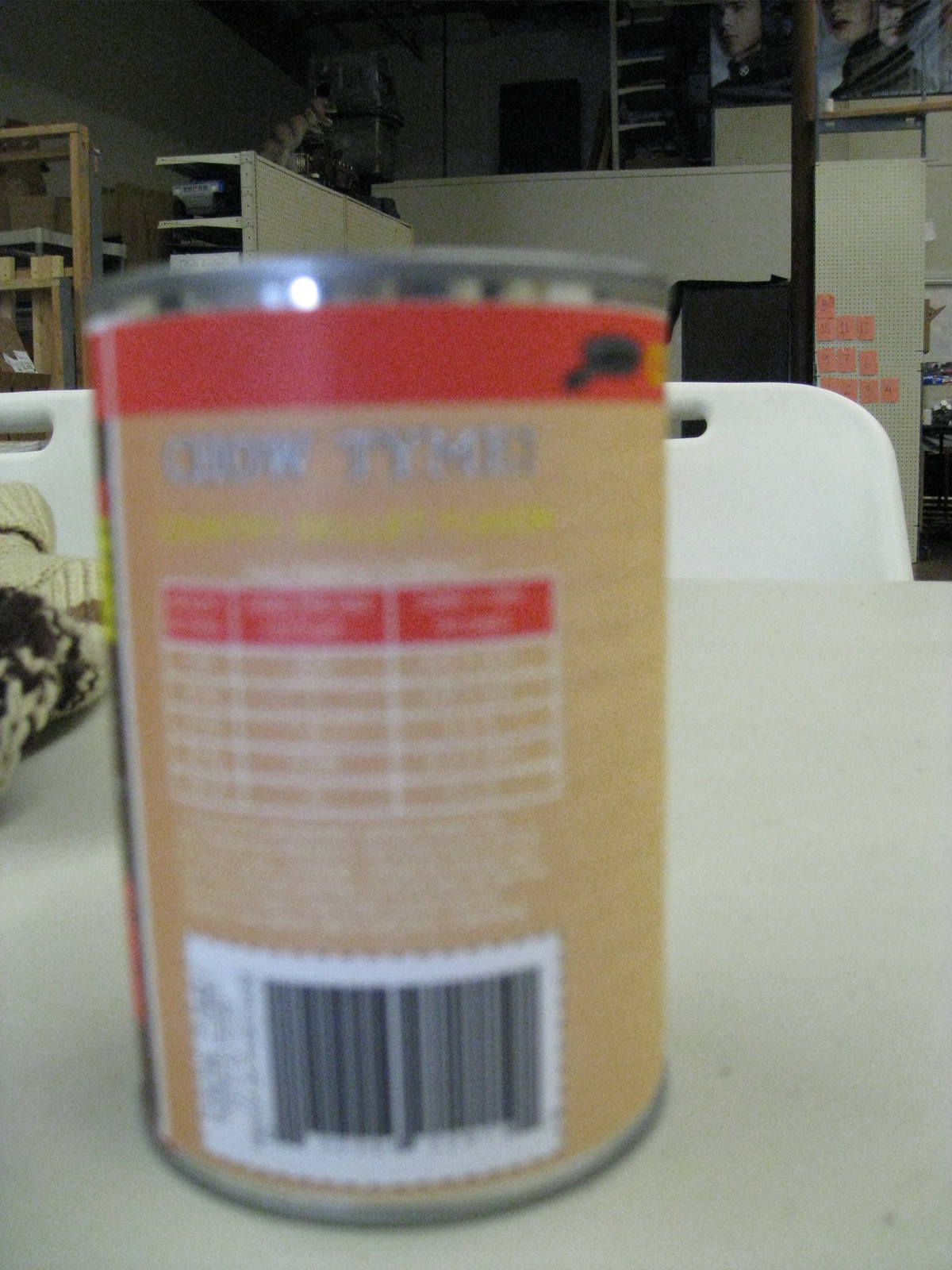In this photograph, a can, predominantly tan and red with splashes of yellow writing, sits slightly blurred on a white table. The can's label, featuring nutritional facts and a barcode at the bottom, is barely readable. The setting appears to be inside a storage container or warehouse, evidenced by the miscellaneous items in the background. Two white chairs are placed near a wall, alongside a ladder. Behind the chairs are two posters, depicting a man and a woman, though the woman's head is cropped out, only revealing her features from the nose down. Additionally, a shelf holding a small T-Rex or dinosaur statue is situated behind the can. Pink lettering is visible on a wall adjacent to the chairs, adding a splash of color to the setting.